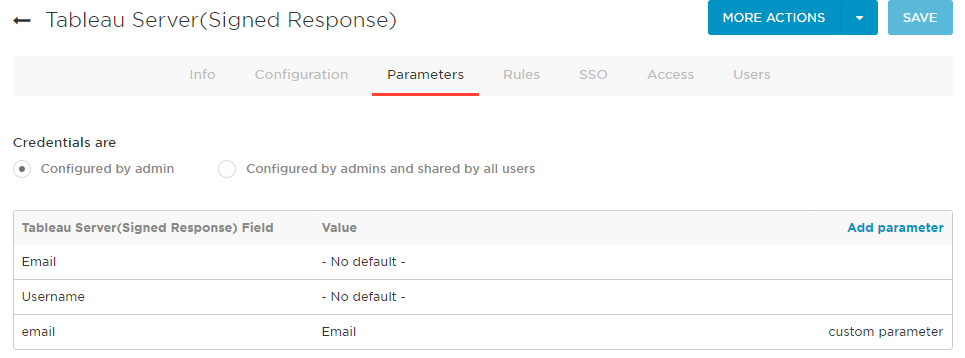**Tableau Server Signed Response Configuration Page**

The image showcases a web page titled "Tableau Server Signed Response," as indicated in the upper left-hand corner in a black font. A black arrow pointing to the left is situated next to the title, all set against a white background. In the upper right corner, there is a pull-down menu labeled "More Actions" with a blue box surrounding it and white font inside. Next to it, also enclosed in a blue box with white text, is a "Save" button.

Below this upper section, a series of tabs are visible, including "Info," "Configuration," "Rules," "SSO," "Access," "Users," and "Parameters." The "Parameters" tab is currently selected, indicated by a red bar underneath it.

The main body of the page begins with the heading "Credentials are" in the upper left. Beneath this heading are options with checkboxes for "Configured by Admin" and "Configured by Admins and Shared by All Others.” The checkbox next to "Configured by Admin" is currently ticked.

Further down, a table is presented with the top row labeled "Tableau Server Signed Response Field" on the left, "Value" in the middle, and "Add Parameter" on the far right, the latter of which is in blue text. Subsequent rows in the table are labeled "Email," "Username," and another "Email."